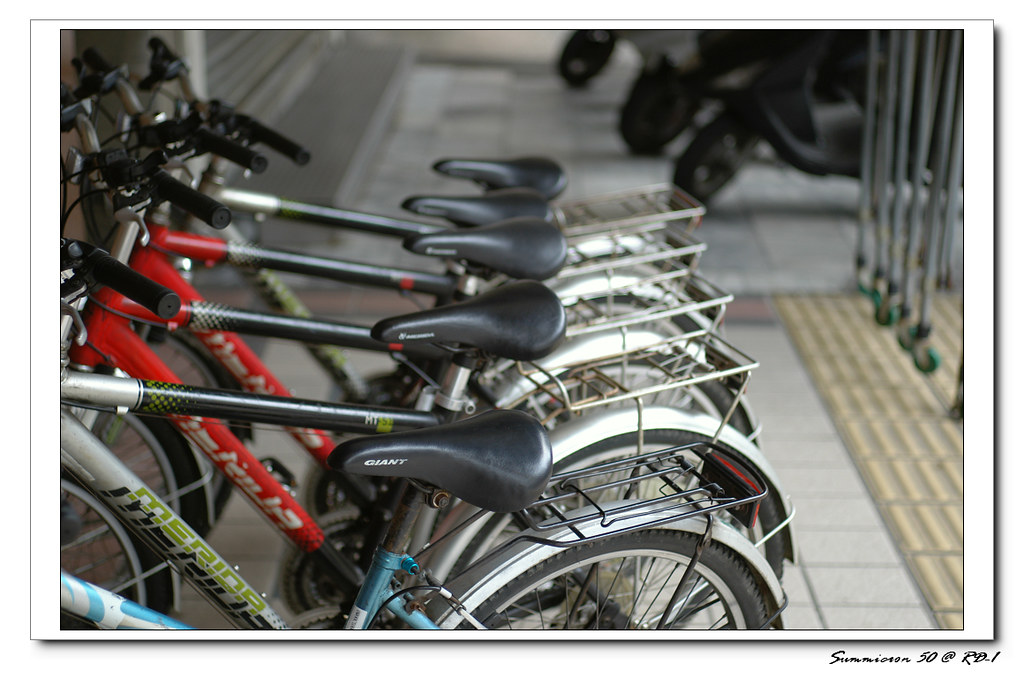The image depicts a professionally composed color photograph featuring a row of five neatly aligned bicycles parked in a bike rack. Each bicycle showcases distinct down tube colors, including blue, silver, and red, but they all have uniform black handlebars, seats, and black wheels with stainless steel fenders. The bicycles also feature steel rear racks and small wire baskets attached above the back tires. The scene is set on a gray stone sidewalk that contrasts with the variety of bicycle colors. In the blurred background, there are additional riding instruments, likely scooters or smaller motorcycles, identified by their smaller tires compared to motorcycles. Hanging down to the right of the image is an indistinct object with wheels, possibly indicative of an enclosure. The photograph has text along the bottom right corner, reading "Simeonsen 50 at RD," which might be the artist's signature.